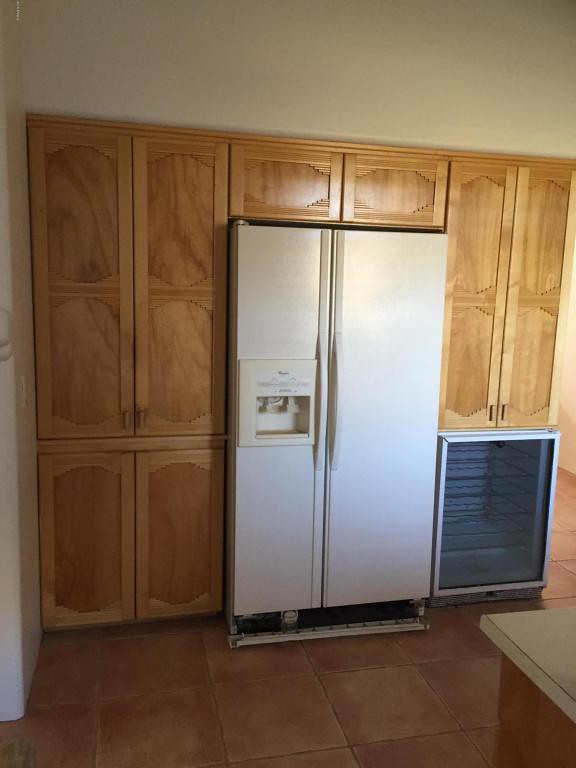The photograph captures a kitchen scene dominated by a built-in side-by-side white refrigerator with an ice and water dispenser on the left door. The refrigerator is seamlessly integrated into a large expanse of natural-finished, blonde wooden cabinetry, which includes enclosed upper cabinets extending above it. To the right of this setup is a half-height wine refrigerator with a clear door, currently empty. The kitchen floor is tiled with large beige tiles, and a portion of a white countertop and another cabinet are visible across the room. The cabinetry and refrigerator unit are set against a beige background wall, creating a cohesive and unadorned aesthetic in the kitchen.